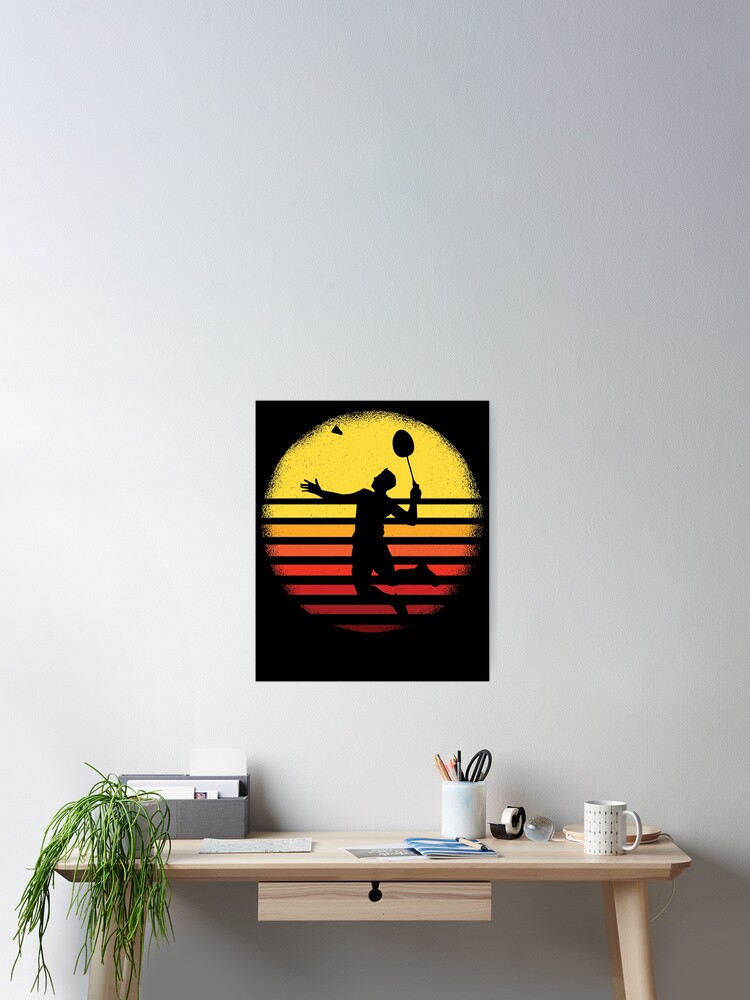This color photograph captures a minimalist desk setup against a stark white wall. Centered above the light wood desk is a small black poster featuring a silhouetted man jumping to play badminton against a yellow sunset with orange bands and vertical black stripes. The desk itself is simple, comprising a single small drawer and resting on four round legs. Atop the desk sits a stringy green plant in a white pot, a gray organizer with unseen documents, and a white swing-arm lamp. Additionally, there is a stainless steel box holding cards, a pencil cup containing pencils, pens, and scissors, as well as a white coffee mug with a gray geometric print. Flanking the left side of the plant is a roll of tape, and tucked in the corner, there are greeting cards. Overall, the desk is compact and utilitarian, suitable for a neat and efficient workspace.